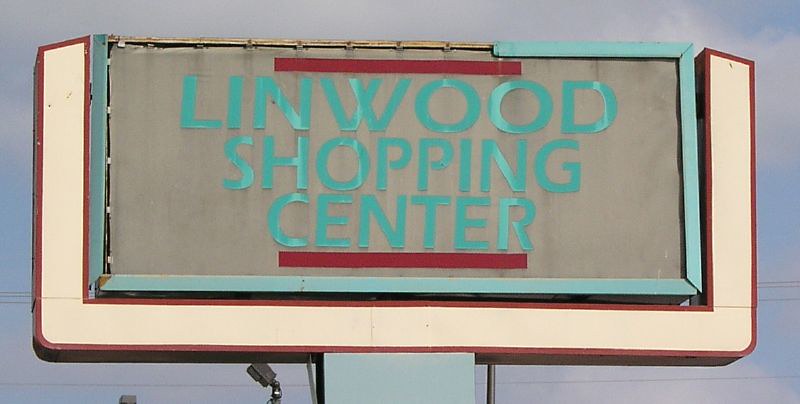The photo features a sign for "Linwood Shopping Center," though the sign appears dilapidated and weather-worn. The rectangular sign, framed in a beige border followed by maroon and green borders, is topped and bottomed with maroon bars. The centerpiece, in a faded light gray, displays the shopping center's name in large blue letters. The top left edge of the blue metal frame is missing, exposing screws, hinting at its age and disrepair. The sign is held aloft by a tall, rectangular turquoise pole. Above and behind the sign, a cloudy sky with patches of blue peeks through, adding to the sense of neglect and abandonment.